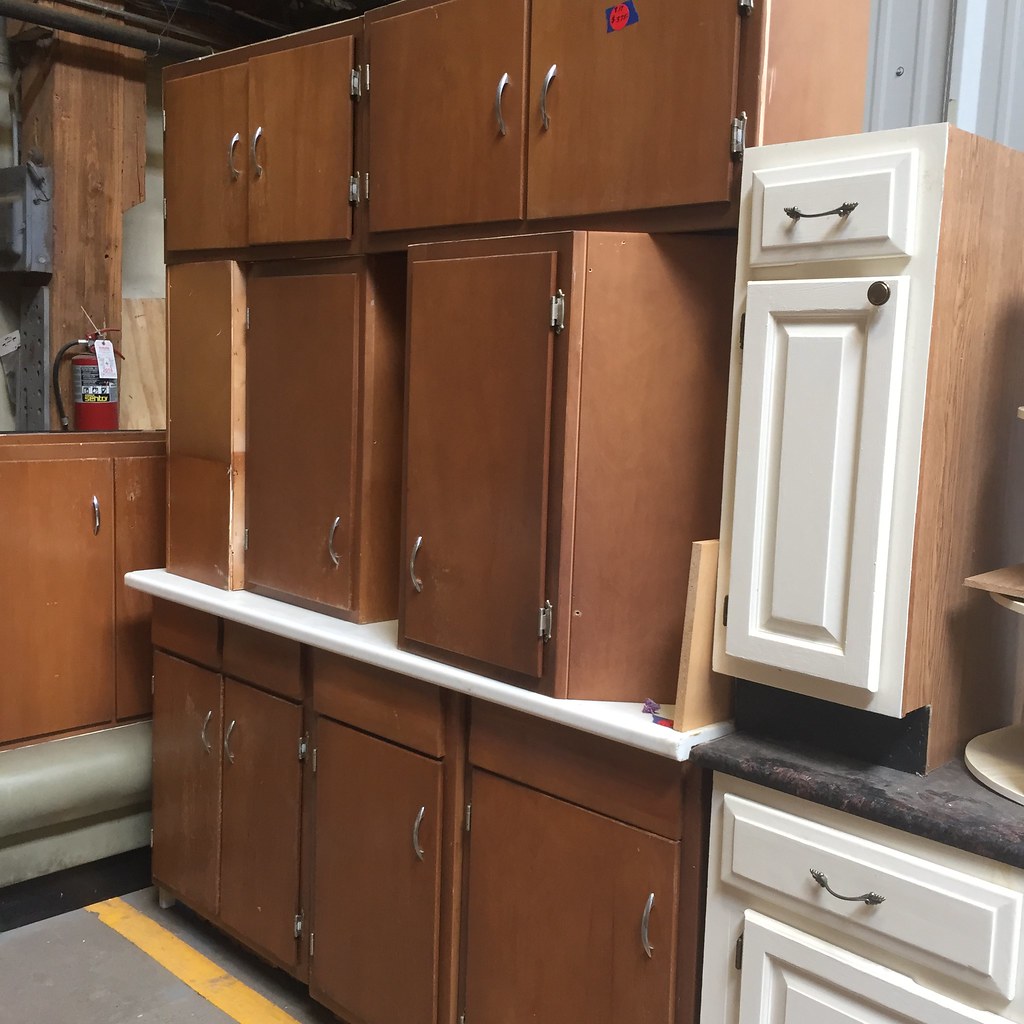The image depicts an arrangement of kitchen cabinetry, likely situated in a showroom, warehouse, or store. The cabinetry primarily features a flat, medium-brown finish with minimal texture. These cabinets are arranged across three distinct levels: the top level showcasing two horizontal sets of cabinets, the middle level comprising three individual units, and the bottom level including four cabinets with smaller drawers positioned above them. Each unit is adorned with sleek, silver handles that curve gently.

On the right side, there is a smaller section of white cabinetry exhibiting a varied design. This includes a small drawer atop a narrow, taller cabinet, which is followed by another cabinet at the bottom, featuring different handle styles and a circular knob. A price sticker is visible at the top of the image, although the details are unreadable. The background includes additional pieces of wood, a red fire extinguisher, and a metallic floor marked with a yellow line, providing an industrial context to the setting.